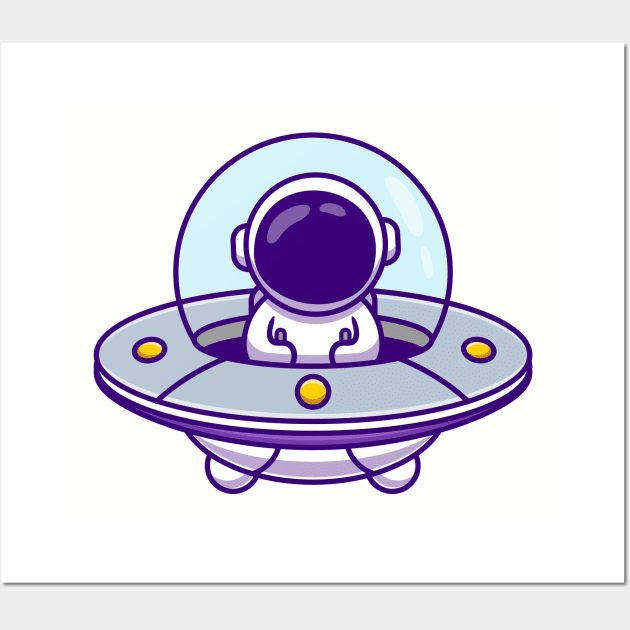This cartoon-style illustration depicts an astronaut inside a small, round UFO-like spaceship, detailed with purple and white colors and gray segments. The spaceship is topped with a large, circular, clear dome, inside which the astronaut is visible, wearing a white space suit and a large round helmet with a dark blue, tinted visor obscuring his face. He is gripping two controls, demonstrating a focused demeanor. The base of the spacecraft is shaped like a bowl, featuring two small landing feet and three yellow lights dotting its surface, adding to its otherworldly charm. The compact design of the spaceship suggests it is meant for only one occupant, emphasizing its intimate and personal scale.